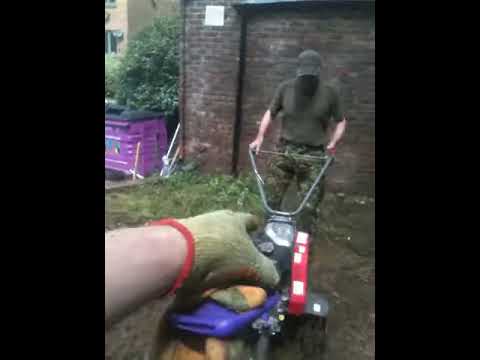In the image, you see a man operating what appears to be a red and black rototiller in an outdoor setting. At the front of the frame, there's an oversized gloved hand, likely due to the perspective, pointing towards the rototiller. The glove is olive green with red trim. The man in the background is wearing a ball cap, a green or gray shirt, camouflage pants, and possibly a face mask. He is gripping the silver handlebars of the rototiller, standing in an area with green grass and patches of dirt being tilled. Behind him is a large dark red brick wall, and off to the side is a purple container, likely used for lawn storage or tools, with a bush growing above it. Additionally, several hand tools are scattered nearby. The image appears to be low resolution with significant compression, making the details somewhat unclear.